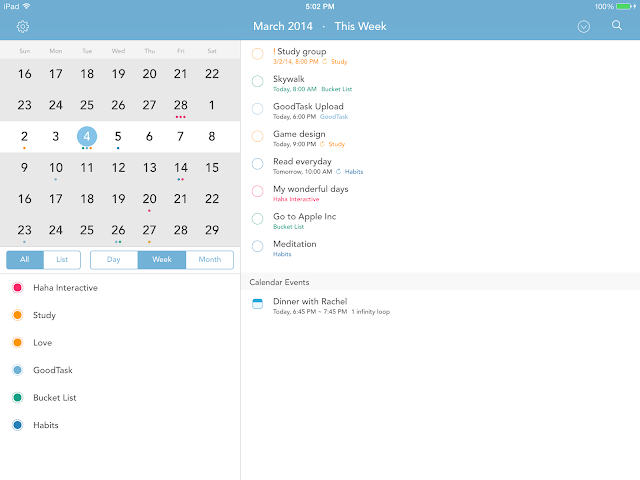The image portrays a detailed and organized digital calendar interface on an iPad screen. In the top left corner, the iPad's Wi-Fi signal icon is prominently displayed, accompanied by a cogwheel symbol to access the device's settings. The blue banner spanning across the top of the screen features the current time, displayed as 5:02 PM, and the date, marked as March 2014, with a note indicating "this week." 

On the right side of this banner, a green-colored 100% battery indicator is visible alongside a magnifying glass icon, suggesting a search function. Directly below the banner, a monthly calendar layout is presented, starting from Sunday and ending on Saturday. Notably, the date 4th is encircled in blue, indicating a special highlight.

To the right of the calendar section, a list of planned activities for the day unfolds. These activities include a study group, a skywalk, a task upload reminder, game design work, daily reading, personal reflections titled "My Wonderful Days," a visit to Apple Incorporated, and a session of meditation, among others.

Beneath the listing of activities, the interface categorizes calendar events with a column of colored dots, each representing different categories: red for "Haha Interactive," orange for "Study" and "Love," blue for "Good Task," green for "Bucket List," and blue again for "Habits."

Overall, the scene captures a meticulously organized daily agenda designed to help the user maintain productivity and balance in their activities.